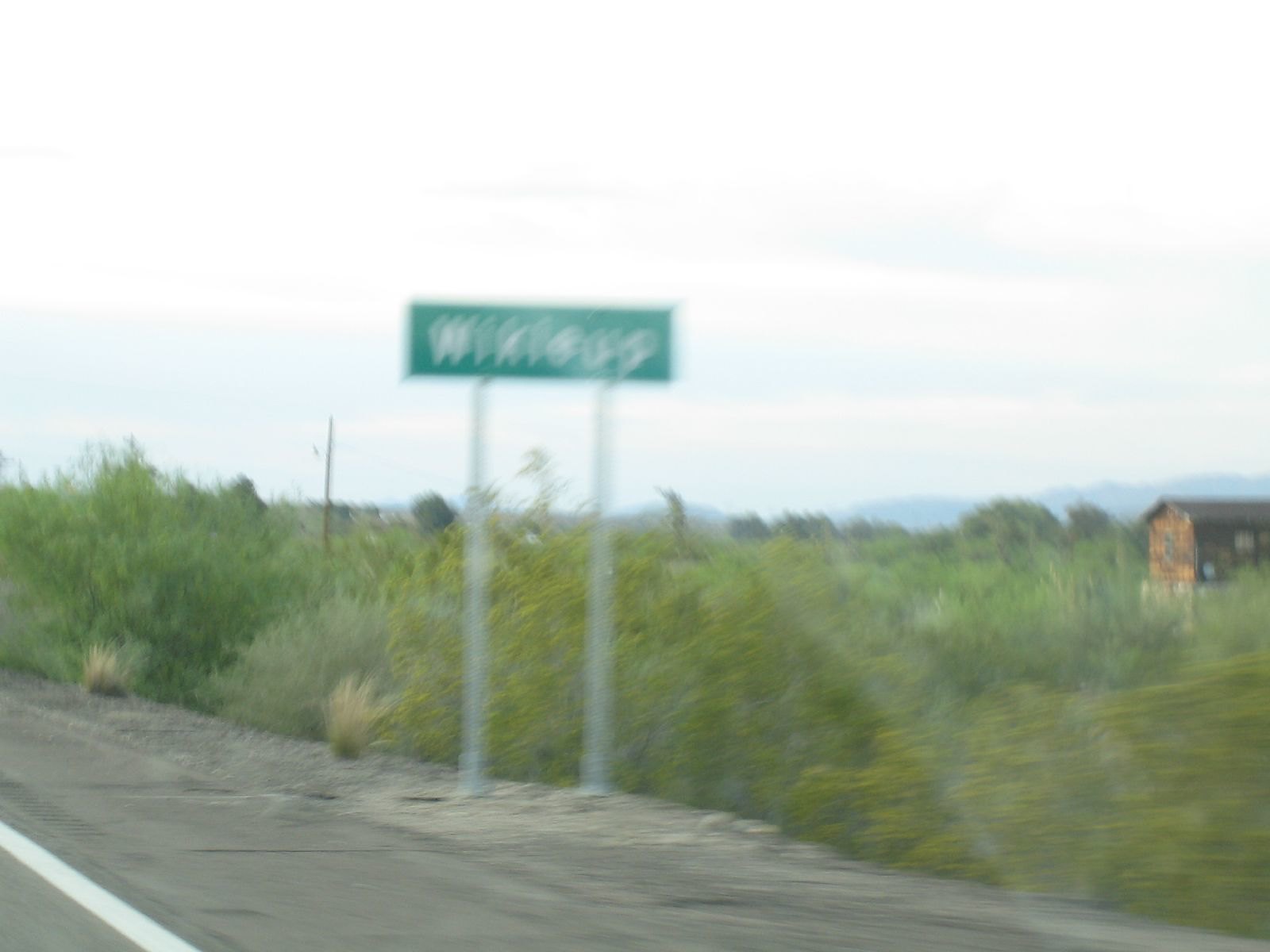This photograph, captured from a moving car, exhibits a blur that suggests motion. The image includes a small, green street sign adorned with white lettering, which is unfortunately unreadable due to the blurriness and angle. The sign is mounted on horizontal silver supports and is positioned on the shoulder of the road, delineated by a solid white line. Surrounding the sign is a patch of tall wild grass and numerous weeds, some of which tower directly behind it. To the right side of the frame, a brown house is partially visible, featuring a couple of windows and what appears to be a fence, although the exact details remain indistinct due to the perspective.